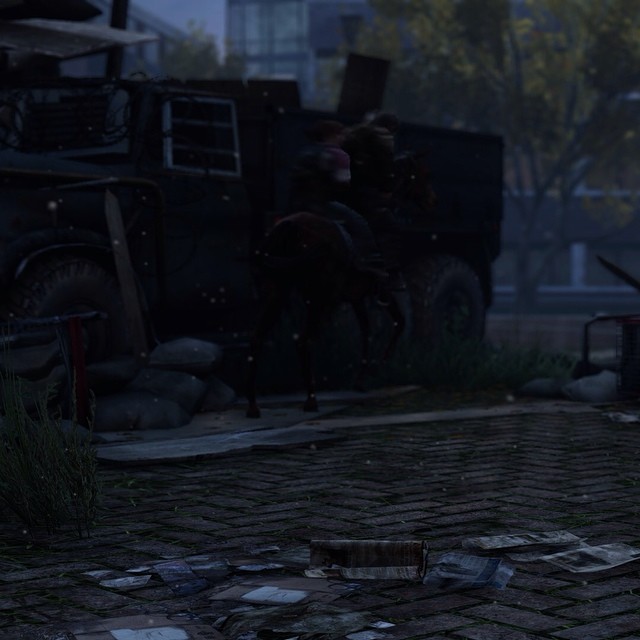The photograph captures a dark and foggy scene, reminiscent of a realistic video game environment set at night. The dimly lit image features tiny white specks floating through the air, evoking an atmosphere of drifting snow or ash. The foreground is dominated by a zigzagged brick sidewalk strewn with old newspapers and magazines. In the center, a man is seated on a horse, both of which appear slightly blurry. The horse, facing away from the camera, allows a partial view of its face and side. The man atop the horse is dressed in dark clothing, possibly overalls.

Behind them, an old wooden wagon with large wheels rests on a patch of grass, flanked by what seem to be stones or large bags. To the left of the wagon stands a pile of grey stones and some kind of metal tool or device. The background reveals a tree with orange leaves, adding a touch of color to the otherwise somber scene. An obscured, large vehicle—perhaps a dump truck—lurks in the background, further hinting at an intricate and layered environment.